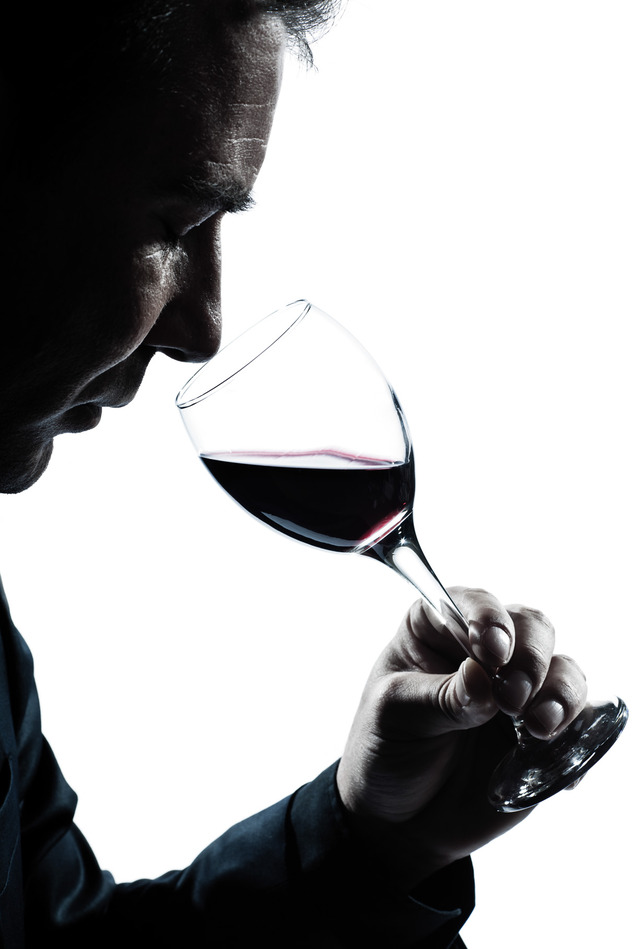The artistic black and white photograph, set against a completely white background, captures a refined moment of a middle-aged man, likely in his 40s or 50s, deeply engaged in the evaluation of a dark-colored wine. Positioned in the top left of the image, his partially visible face, with closed eyes, suggests a focused, sensory examination. The man's left hand, emerging from a long-sleeved garment, elegantly holds the stem of the glass between his thumb, index, and middle fingers, with his pinky gently supporting the base. The wine swirls slightly, filling the glass to about halfway. The minimalistic composition and subtle lighting emphasize the contemplative nature of this wine connoisseur, giving the photograph a near-silhouetted effect while still allowing the man’s facial features and the faint blue hue of his shirt to be discerned.